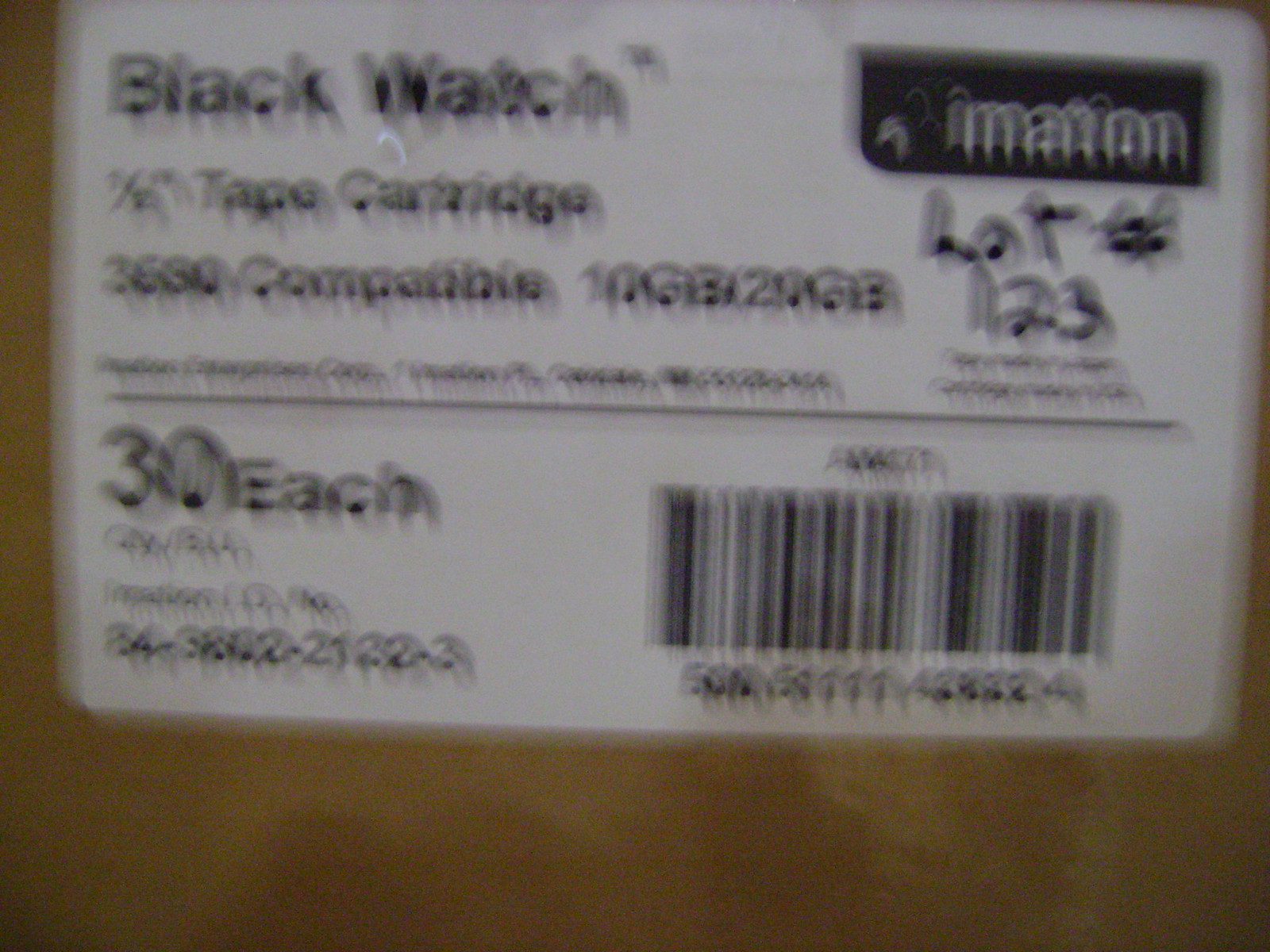This is a somewhat blurry photograph of a cardboard box featuring a distinct white and black label. Despite the blur, the label reveals key details. The box is from the Imation brand and prominently displays the text "Black Watch" at the top in black font. The label indicates it contains half-inch tape cartridges that are 3660 compatible, with storage capacities noted as 10 gigabytes and 20 gigabytes. The quantity is marked as 30 each. A barcode is visible at the bottom right, accompanied by some numbers that are partially obscured by the blur. Additionally, there is a handwritten lot number "123" inscribed in black marker. The label also includes some smaller, unreadable text due to the blur, and towards the bottom of the image, the box features a darker colored portion.